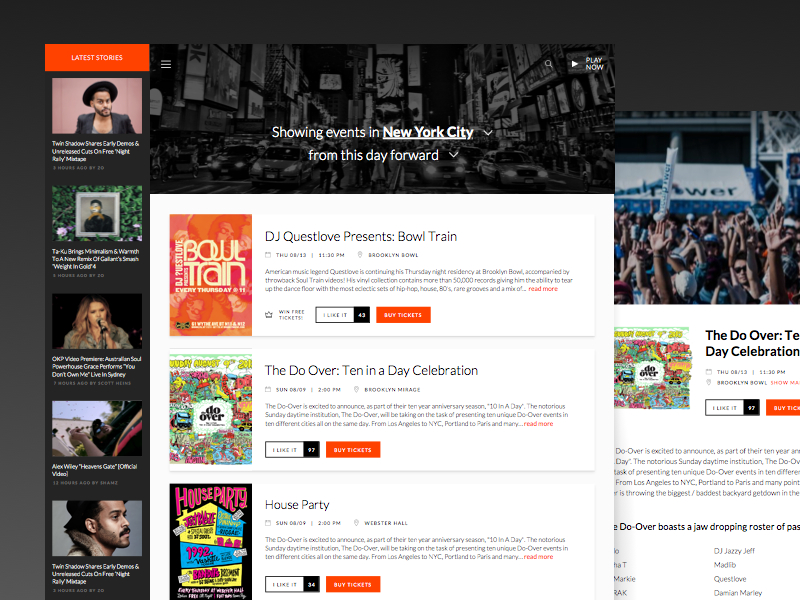**Event Highlights in New York City**

In the bustling top section of the main page, a black pop-up features a striking black-and-white image of Times Square. Prominent white text announces "Showing events in New York City," with "New York City" underlined and accompanied by a downward white arrow.

Moving down, the text "From this day forward" with a similar downward arrow guides the eye to the prompt "Play Now." The background then transitions to white, introducing a bold black announcement: 

**DJ Questlove Presents: Soul Train**
- *Platform:* Brooklyn Bowl
- *Date:* Thursday, August 12
- *Time:* 11 p.m.

American music legend Questlove continues his Thursday night residency at Brooklyn Bowl, igniting the dance floor with classic Soul Train videos and a curated selection from his Rhino vinyl collection, which boasts over 50,000 records. Expect an eclectic mix of hip-hop, house, 80s rarities, and more. [Read More]

Beneath this announcement, two interactive boxes are visible:
1. A black-and-white box stating "I like that"
2. A red box urging "Buy Tickets"

**The Do-Over: 10th Anniversary Celebration**
- *Dates:* Upcoming Sundays
- *Time:* 2 p.m.
- *Venue:* Brooklyn Mirage

Celebrating 10 years, the Do-Over will host their iconic Sunday daytime parties across 10 cities, including Los Angeles, New York City, Portland, and Paris. Each city will feature unique events under the theme "10 in the Day." [Read More]

**House Party**
- *Venue:* Webster Hall

Notably overlapping in date and time with the previous event, this entry reiterates the excitement of simultaneous celebrations at renowned venues across New York City.

Take action now by exploring these events further and securing your tickets to join in on the musical festivities.